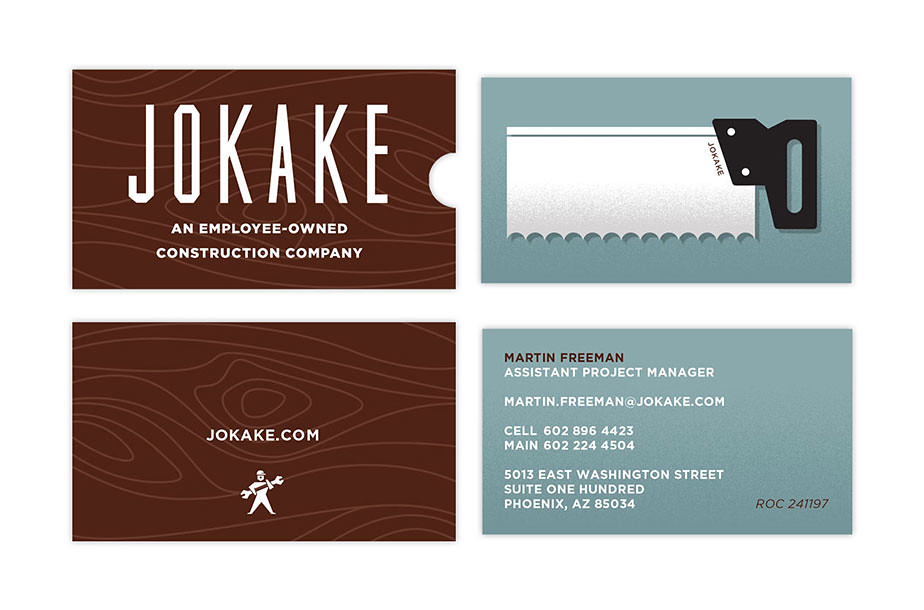The image showcases a design mock-up that includes two sets of business cards and their corresponding sleeves. Each sleeve and card design features distinct elements but shares a cohesive theme centered around the brand "Jokake".

The top left quadrant displays the front of a business card sleeve. It has a maroon background with light maroon, wood grain-like lines. Prominently featured in large white text is "JOKAKE," and below it, in smaller white text, "An Employee-Owned Construction Company." The corresponding back of the sleeve (bottom left) continues the maroon theme and centrally displays the URL "JOKAKE.COM" in small white letters. Below this, there's an illustration of a construction worker holding an oversized wrench, adding a whimsical touch. The sleeve also has a semi-circle cut-out along one edge.

On the right side, the upper right quadrant shows the front of a business card against a blue background. It features an illustration of a hand saw with a black handle, displaying the name "JOKAKE" on the blade. The back of this card (bottom right) lists detailed contact information against the same blue background. "MARTIN FREEMAN" is prominently displayed at the top in black text, followed by his title, "Assistant Project Manager," along with his email "MARTIN.FREEMAN at JOKAKE.COM". Further down are the contact numbers: cell (602-896-4423), main (602-224-4504), and the office address: "5013 East Washington Street, Suite 100, Phoenix, Arizona 85034." The bottom right corner of this section notes the ROC number "241197."

Together, these elements provide a comprehensive and detailed visual identity for Jokake, blending professional information with creative, industry-relevant illustrations.